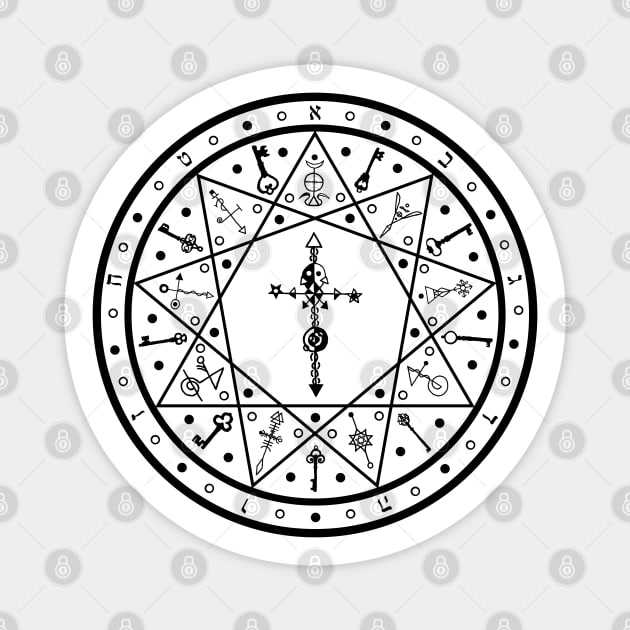The image features a detailed and intricate design set against a simple grey and white dotted background with prominent watermarks resembling white lock icons. At its center lies a large white circle containing a complex, pentagram-like figure nestled within multiple concentric black circles. This primary black circle contains an elaborate array of symbols including tarot-like imagery such as keys, moons, black circles, and dots, giving the image a slightly cultish but captivating feel.

The central emblem or design exudes qualities of a compass or a circled pattern. It combines a multitude of symbols: keys of various shapes, a crust-like feature, and alternating black and white dots that emphasize the detailed nature of the emblem. Every fourth dot contains a unique symbol, some resembling musical keys or the mathematical symbol for pi, adding to the complexity of the design. The pentagram-like star figure itself is constructed of intersecting triangles, contributing to the layered and intricate appearance of the entire image.